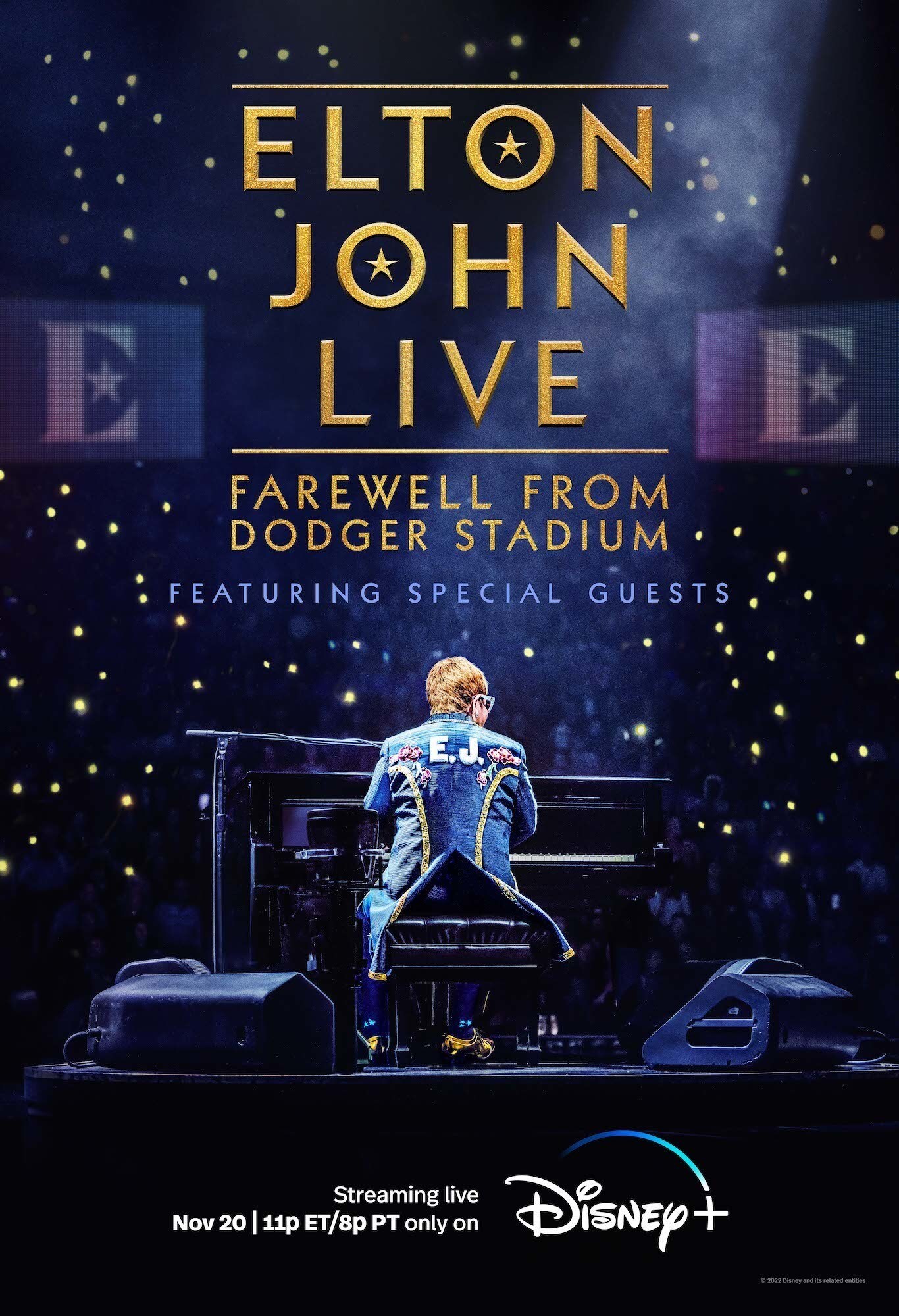**Descriptive Caption:**

In a visually striking advertisement, "Elton John Live" is prominently displayed across three lines, with the 'O' in "Elton" and 'O' in "John" creatively designed to feature a star. This headline is accentuated by two dividing lines, one above and one below, separating it from the secondary text, which reads "Farewell from Dodger Stadium" in a luxurious gold font.

Below this, in contrasting blue text, it announces "Featuring Special Guests." The image captures Elton John himself, adorned in a dazzling blue coat and seated gracefully on a black chair in front of a matching black grand piano. His brownish hair adds to his distinguished appearance, and his coat is emblazoned with "EJ" in white on the back. He is poised on a sleek black platform, surrounded by the soft glow of myriad red and orange lights from the captivated audience, with some attendees faintly visible.

Above him, a spotlight illuminates the scene, and two large 'E' signs are visible in the background, adding to the concert's majestic atmosphere. The bottom of the advertisement reveals the crucial details in white text, announcing "Streaming Live November 20th 11pm ET / 8pm PT only on Disney+."